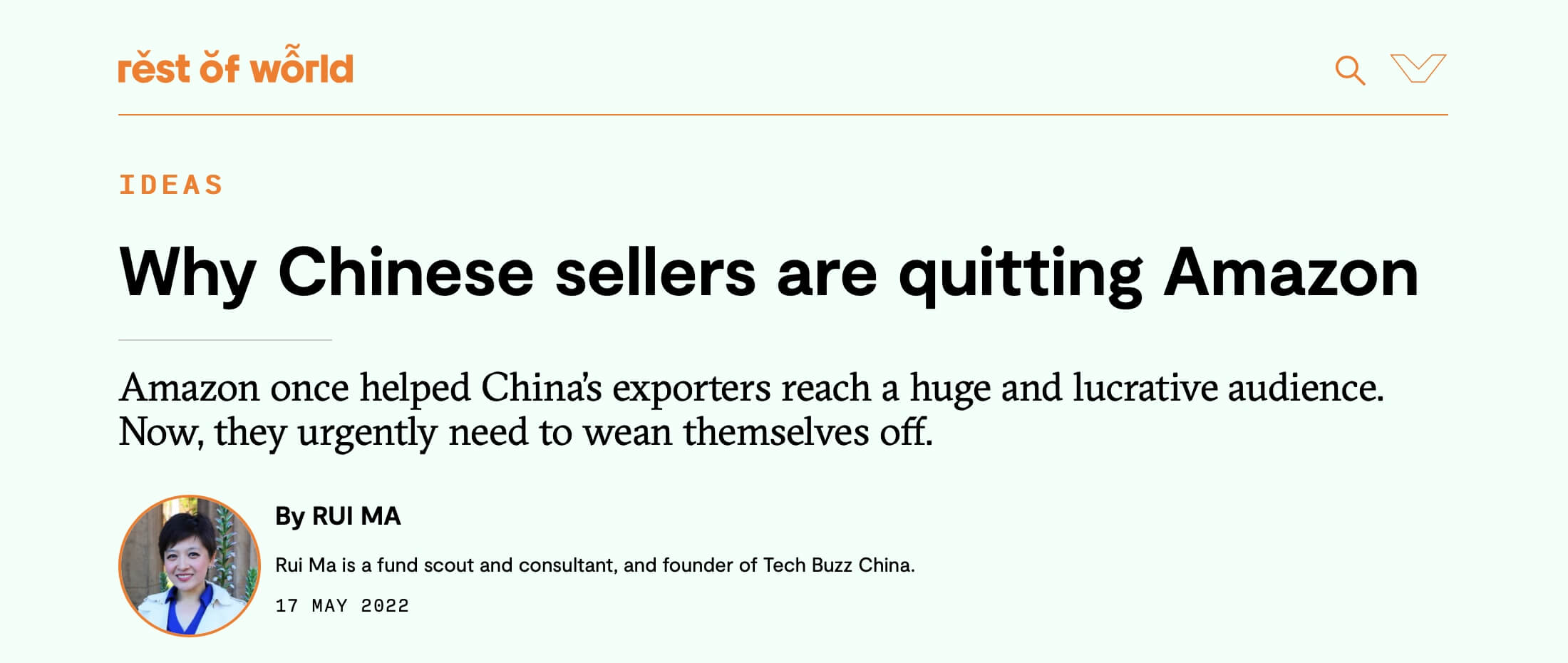This is a screenshot capturing a segment of a website characterized by a clean, white-beige background. The top left corner prominently displays the text "Rest of the World" in orange font. Notably, there are distinctive marks: a small arrow above the letter 'E', another above the 'O' in "of," and two little swirls above the 'O' in "World". In the top right corner, icons for a magnifying glass and a 'V' are visible. Below this header, an orange line separates the sections.

Further down, the section titled "Ideas" appears in orange font, followed by a headline in large, bold black font that reads, "Why Chinese Sellers Are Quitting Amazon." Below the headline, there is a subtext in smaller black font: "Amazon once helped China's exporters reach a huge and lucrative audience. Now they urgently need to wean themselves off." The article is authored by Ru Ma, and her credentials follow in a smaller font: "Ru Ma is a fund scout and consultant, and founder of Tech Buzz China."

Adjacent to the authorship info is a small circular photo of Ru Ma, who appears to be an Asian woman in her 50s, dressed in a white shirt with a blue collar. The date "17 May 2022" is noted at the end of the block of text.